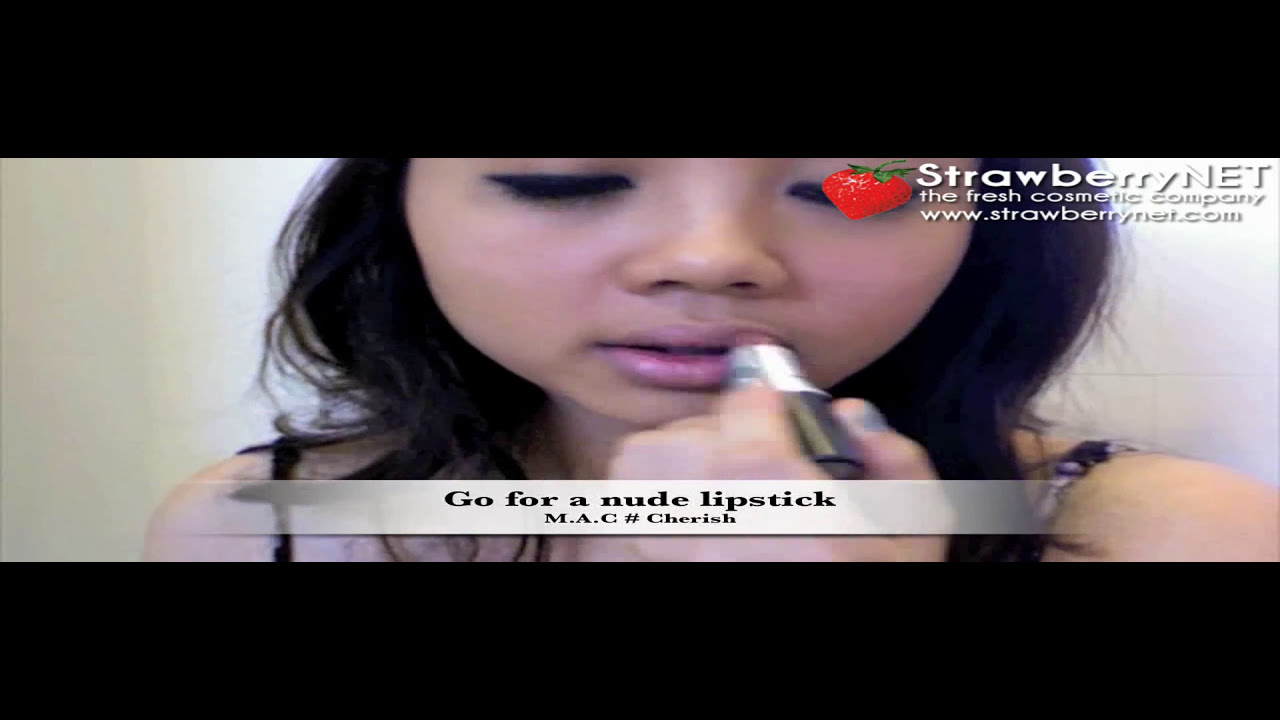The image appears to be an advertisement featuring a young Asian woman standing against a wall. The woman, with long dark hair cascading down both sides of her face, is shown applying lipstick with a black eyeliner on and her eyes closed. She's wearing a shirt with spaghetti straps, and only the top portion of her shoulders is visible. The lipstick she is applying has a brown bottom and a silver middle. 

Across the top and bottom of the image are large black bars, giving the appearance that the image is slightly cropped or squished. In the top right-hand corner, a red-colored strawberry is pictured alongside the text "Strawberry Net, The Fresh Cosmetic Company," with the website "www.strawberrynet.com" below it. Spanning across the middle of the advertisement, there is a somewhat opaque white banner with black lettering that reads, "Go for a Nude Lipstick, MAC #Cherish."